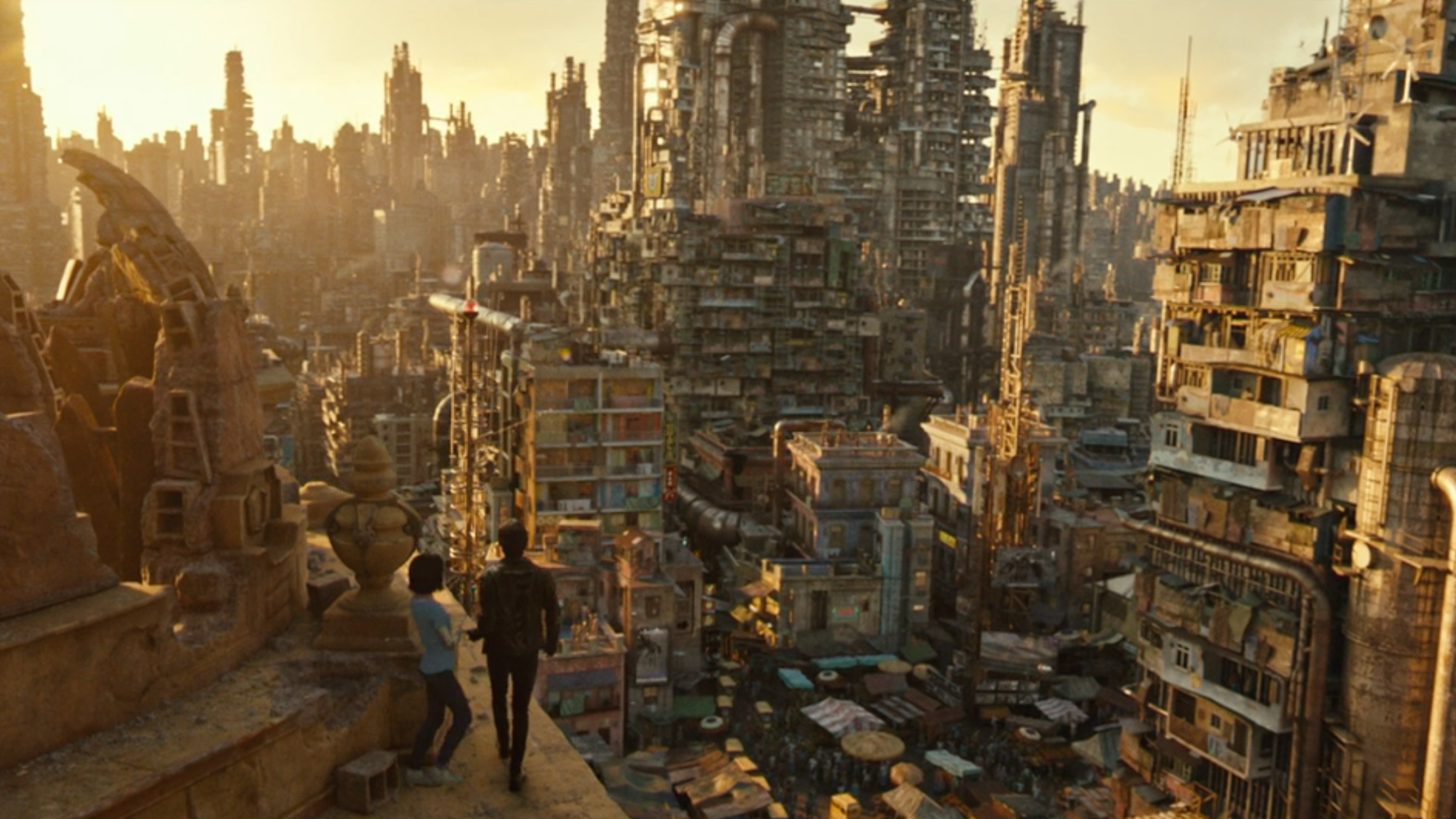A meticulously detailed 3D rendering reveals a scene that could be from an animated film, video game, or digital artwork. In the foreground, standing on a platform, are two stylized characters—a man and a woman—with their backs turned to the viewer. The man, positioned on the right, is dressed in a black outfit, while the woman, standing to his left, wears a light gray top. They overlook a vast, densely populated cityscape that exudes an air of impoverishment and age. The city's buildings are crowded together, appearing old and worn, some adorned with hanging laundry and makeshift planks. Below the platform, the ground level is visible, bustling with activity. Tents are pitched among the throng of figures, adding to the sense of a community making do with limited resources. The intricate details of the setting, from the architecture to the dynamic street life, create a vivid, immersive atmosphere.